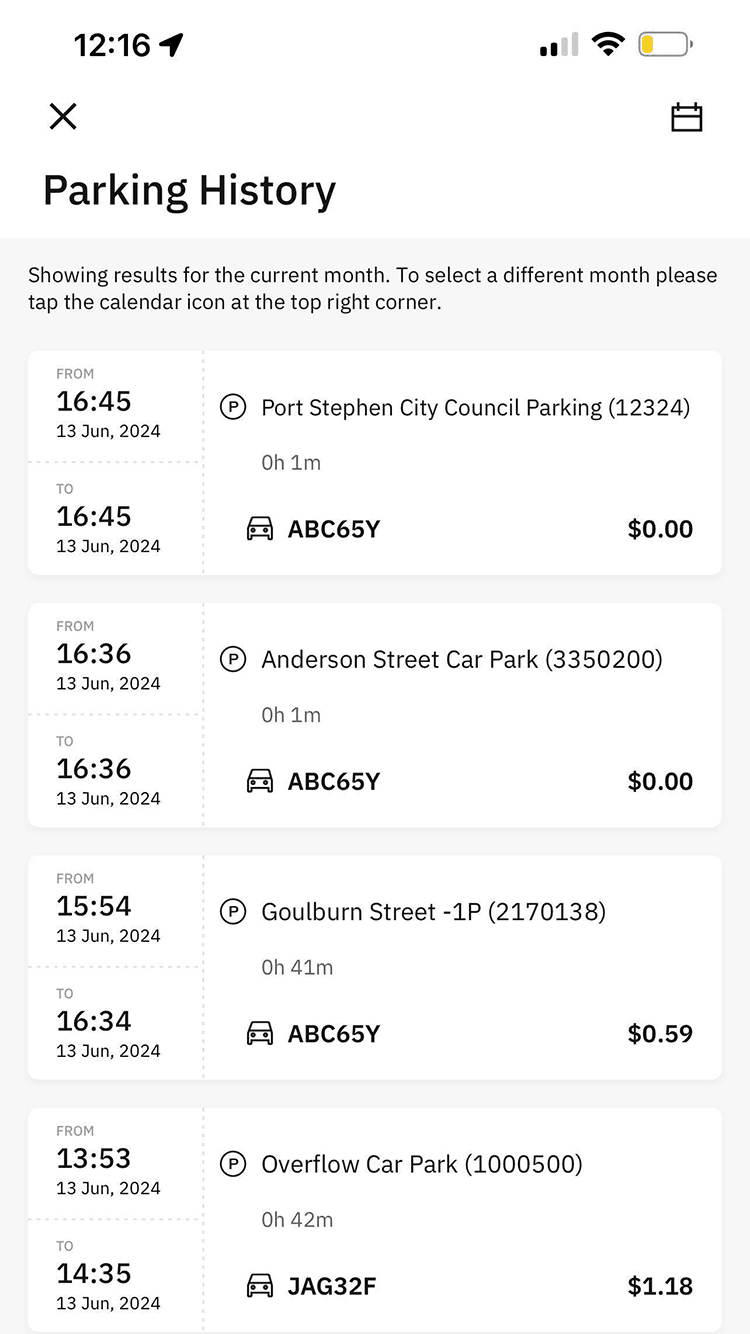The smartphone screen displays a detailed parking history for the current month, including several entries. The time on the phone is 12:16 PM, with two bars of internet connectivity, and the battery level is at approximately 20%. There is an option to view parking history that can be closed by tapping the 'X'. The current screen shows parking details for the current month, with an option to select a different month via the calendar icon at the top right corner.

The parking history entries are as follows:
1. On June 13, 2024, at 16:45 (military time), parked at Port Stephen City Council Parking for one minute with no charge.
2. Nine minutes earlier, at 16:36 on June 13, parked at the Anderson Street Car Park for one minute, also with no charge.
3. On June 13, from 15:54 to 16:34, parked at Goldbloom Street for 40 minutes, incurring a charge of 59 cents.
4. On June 13, from 13:53 to 14:35, parked at the Overflow Car Park for 42 minutes, with a charge of $1.18.

It appears that the individual pays for their parking online through the app.